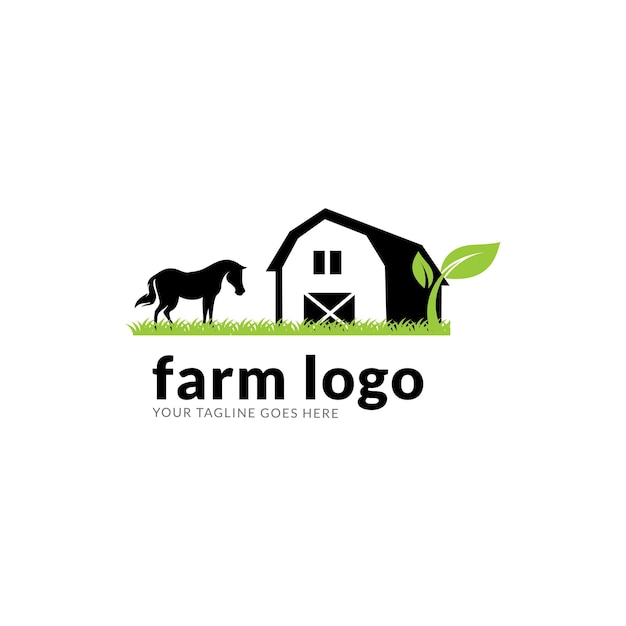The image is a template logo set against a white background, featuring a black silhouette of a horse standing on green grass in front of a barn. The barn, depicted in a simple black and white silhouette style, has a front door marked with a white X and two small black windows above it. To the right of the barn, there's a large green vine with two leaves extending upward. Below the barn and horse, the words "Farm Logo" are prominently displayed in big black lettering, with smaller gray text below that reads "your tagline goes here." This logo template is designed to be customizable, likely sourced from a logo website.